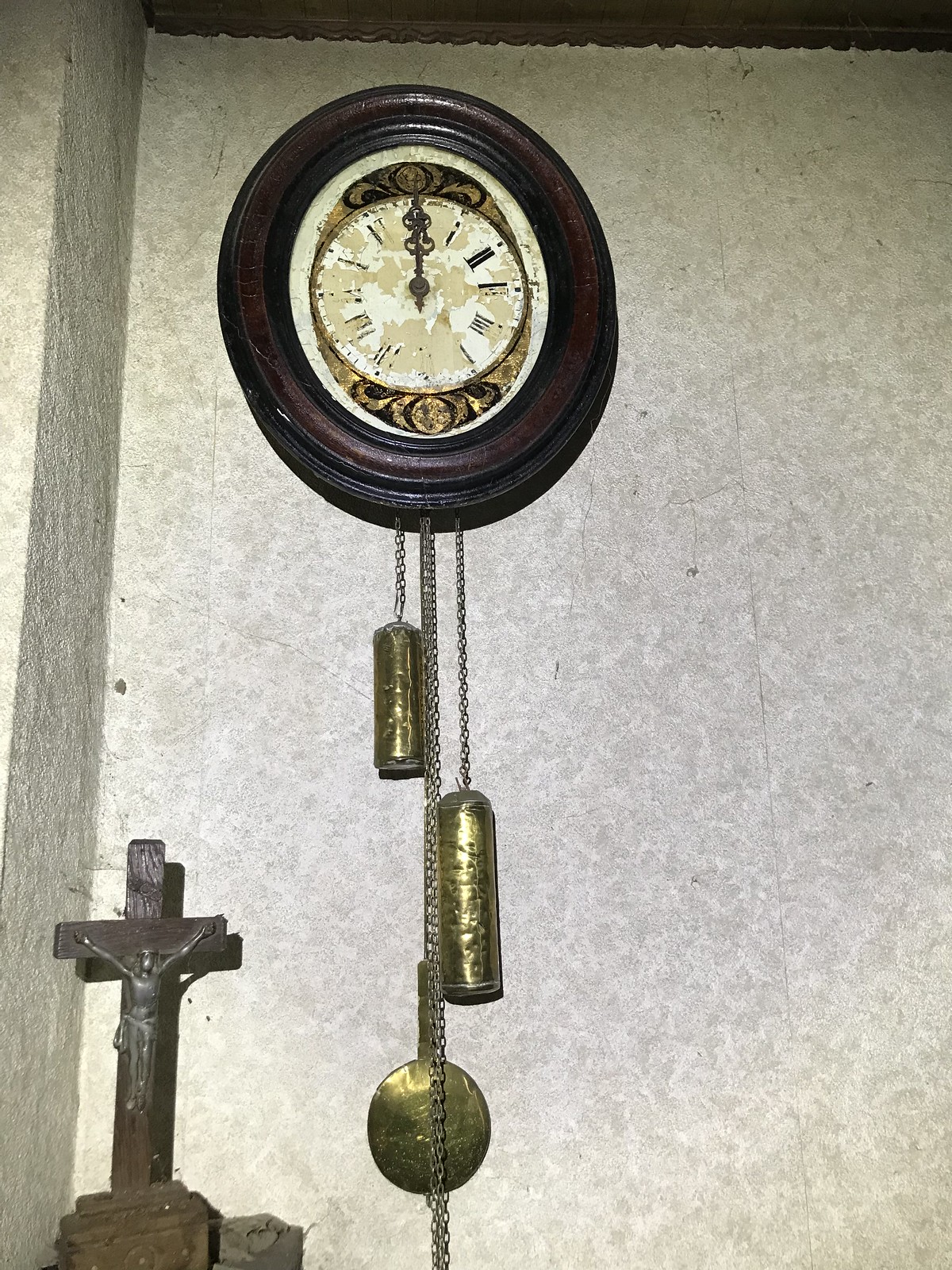This photograph captures a vintage wall-mounted clock with an intricately designed brown, double-layered circular frame. The clock's face features an elaborate globe design accented in gold, adorned with feather-like extensions. The fading and scratched Roman numerals add to the antique charm, while the hour and minute hands, both poised at 12 o'clock, suggest high noon or midnight. The clock includes a pendulum and two bronze-colored weights, both suspended by a lengthy chain, enhancing the overall old-world aesthetic. The clock is positioned on a stark white wall, and beneath it, a bronze-toned crucifix rests gracefully on a shelf, contributing to the timeless ambiance of the scene.